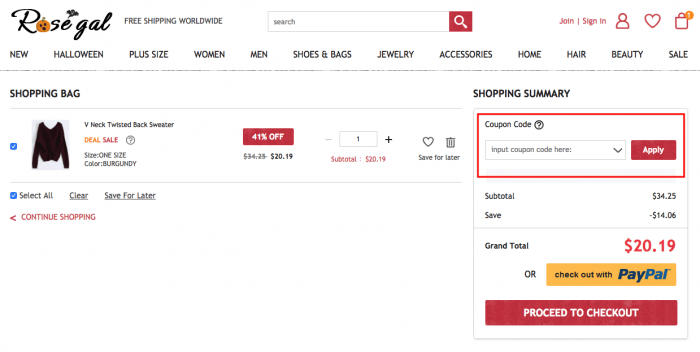This is a detailed view of the desktop page of the shopping website Rosegal. The page has a clean, white background with predominantly black text. At the top of the page, the Rosegal logo is prominently displayed alongside text indicating "Free Shipping Worldwide." A search box is present, and the options to join or sign in are highlighted in red text, accompanied by icons of a person, a heart, and a shopping bag.

Below these elements is a navigation bar featuring categories such as New, Halloween, Plus Size, Women, Men, Shoes & Bags, Jewelry, Accessories, Home, Hair, Beauty, and Sale, likely with drop-down tabs for each. A horizontal bar stretches beneath the navigation menu.

On the left-hand side, the page shows the contents of the shopping bag. An item, a V-neck twisted back sweater, is listed with a tag indicating 41% off, marked in white text on a red rectangle. The quantity of the item can be adjusted, and there are options to save the item for later or remove it using a garbage bin icon.

To the right, a shopping summary is displayed. This section includes fields for a coupon code, a subtotal amount, savings, and the grand total. Below these fields, there are options to pay with PayPal or proceed to checkout.